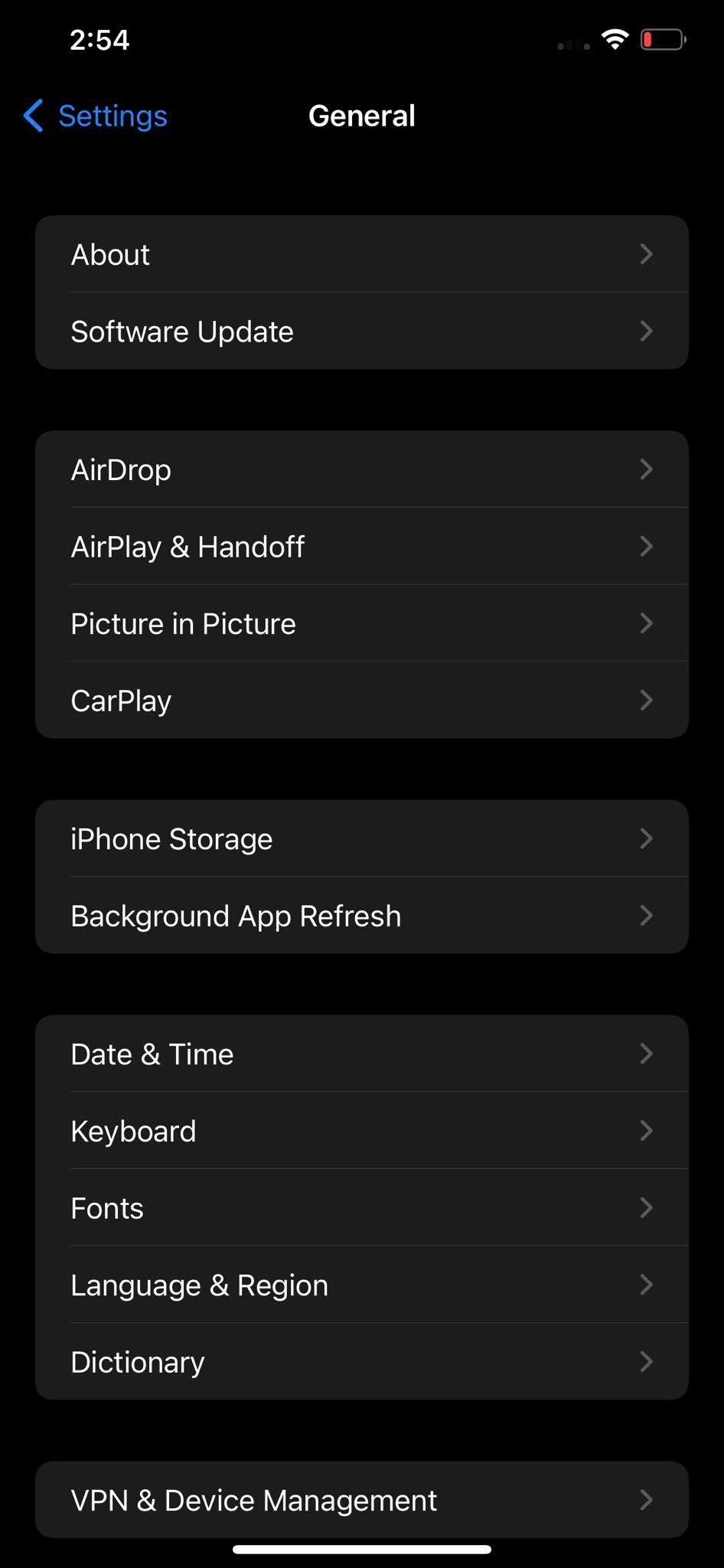The image displays the "General" settings menu for an iPhone, evident from the word "iPhone" and the familiar interface. The background is black, providing a sleek and modern look. At the top of the screen, the word "General" is prominently displayed, confirming that this is the general settings section. The menu lists several options in a vertical format: "About," "Software Update," "AirDrop," "AirPlay & Handoff," "Picture in Picture," "CarPlay," "iPhone Storage," "Background App Refresh," "Date & Time," "Keyboard," "Fonts," "Language & Region," "Dictionary," "VPN," and "Device Management." Each setting is clearly delineated, making navigation straightforward for users seeking to modify their device's settings.